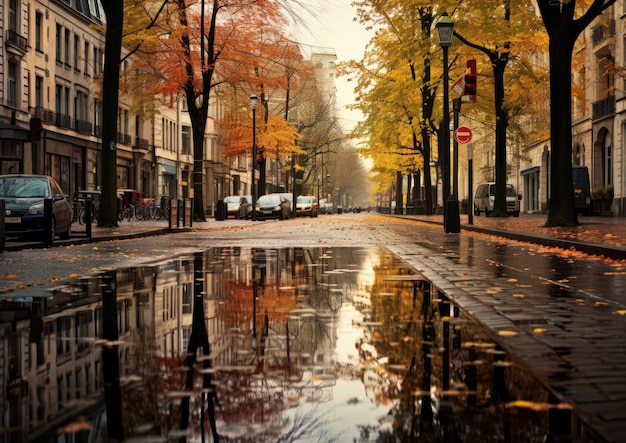The image captures a serene, residential city street in the fall, characterized by tall townhouses and apartment buildings, most likely brownstones with distinctive brick or sandstone facades, arched doorways, and several square windows, some of which host shops or diners with outdoor seating. Lined with big trees adorned in vibrant yellow, orange, and red leaves, the street creates a picturesque autumn scene. The photo, taken from ground level, prominently features a large puddle in the middle of the wet, cobblestone-lined street, reflecting the surrounding buildings and colored foliage. Parked cars and bicycles are seen along the sides of the street, suggesting it's usually a busy area. The street is equipped with old-fashioned streetlights and meters, adding to the charming, old-city ambiance. The overcast sky and setting sun hint that it is late in the afternoon, and the recent rain adds to the serene, slightly melancholic atmosphere of this fall day in the city.